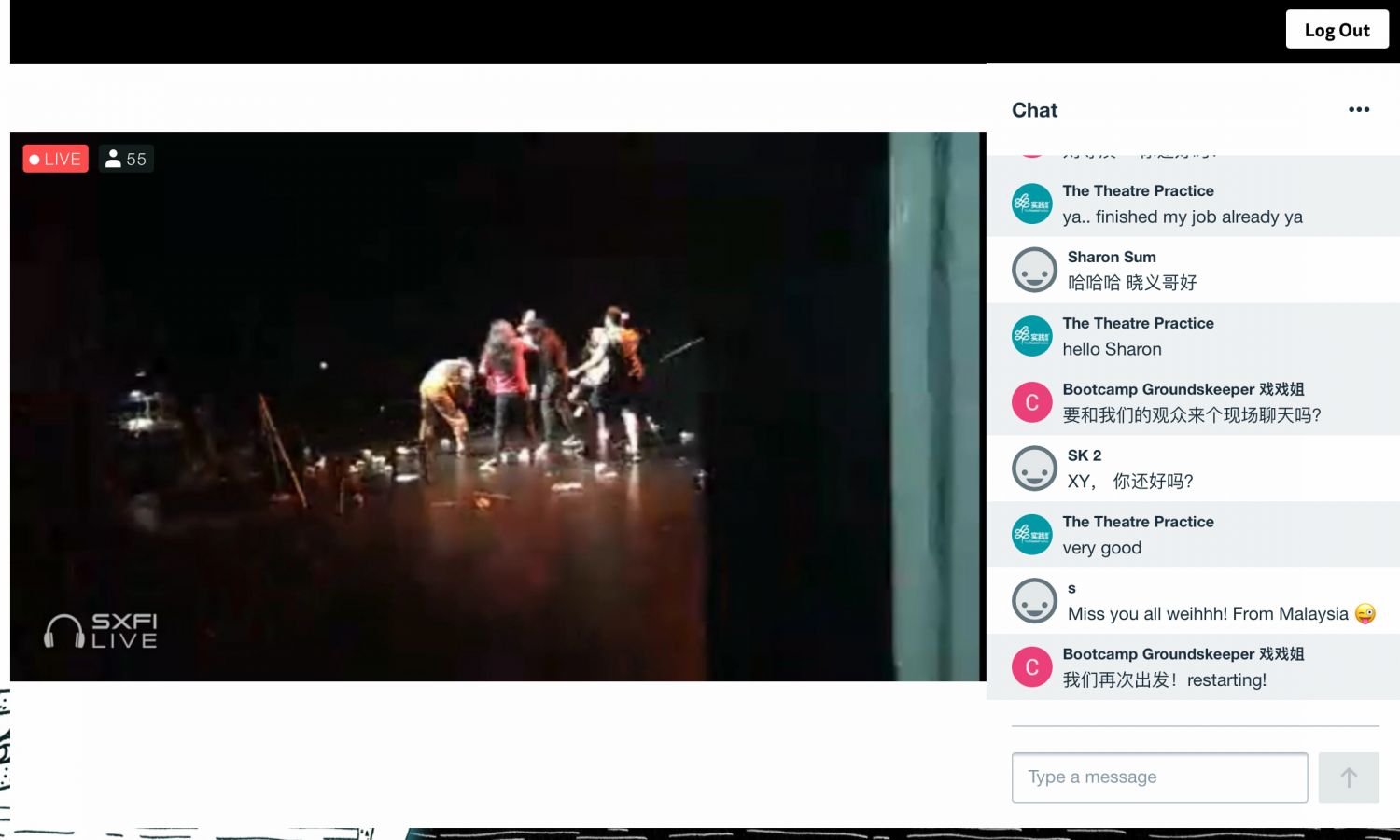This image captures a YouTube live stream interface showing a live broadcast labeled "6x5 Live" in a red box in the upper left-hand corner, indicating it's currently live with 55 viewers. The main content of the live stream is a backstage view of a band performing. The scene is dimly lit, focusing the illumination on the performers on stage. Among them, a man in a red shirt and a woman in a black tank top stand out clearly. 

To the side, there is a live chat section with alternating gray and white boxes where viewers are actively discussing the performance. Various icons in gray, green, and pink accompany the chat messages. At the top of the interface, a long black section features the "Log Out" option in white text. Additionally, there is a section for viewers to type messages, presented in white text, alongside a gray box with an upward arrow. The overall background of the screen is white, providing a clean contrast to the other elements displayed.